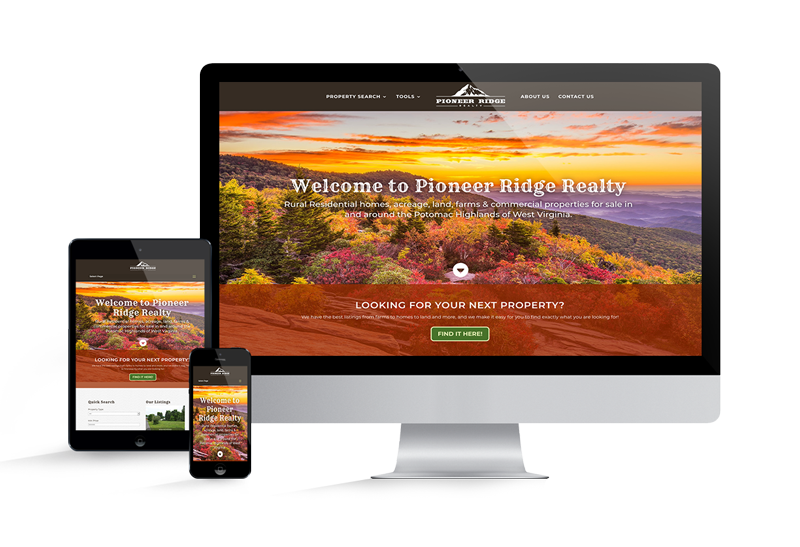The image showcases a monitor, a desktop, an iPad, and an iPhone, all displaying the same screensaver for Pioneer Ridge Realty. At the top of each screen, the website navigation features tabs for "Property Search," "Tools," "About Us," and "Contact Us." The background image is a picturesque scene of a snow-dusted mountain set against a vibrant autumn landscape with trees showing brilliant hues of pink, red, orange, yellow, and light green. To the right, the scene extends to include an ocean under a sky filled with clouds illuminated by a setting sun. The center of the display features a white arrow encircled by a white ring, with the text "Looking for your next property? Find it here," where "Find it here" is highlighted in green with white writing. This vivid and inviting setup is consistently presented across all devices, though the layout is naturally adjusted to suit the smaller screens of the iPad and iPhone. The screensaver encapsulates the essence of Pioneer Ridge Realty, promoting their offerings of rural residential homes, acreage, land, farms, and commercial properties available in the Potomac Highlands of West Virginia.